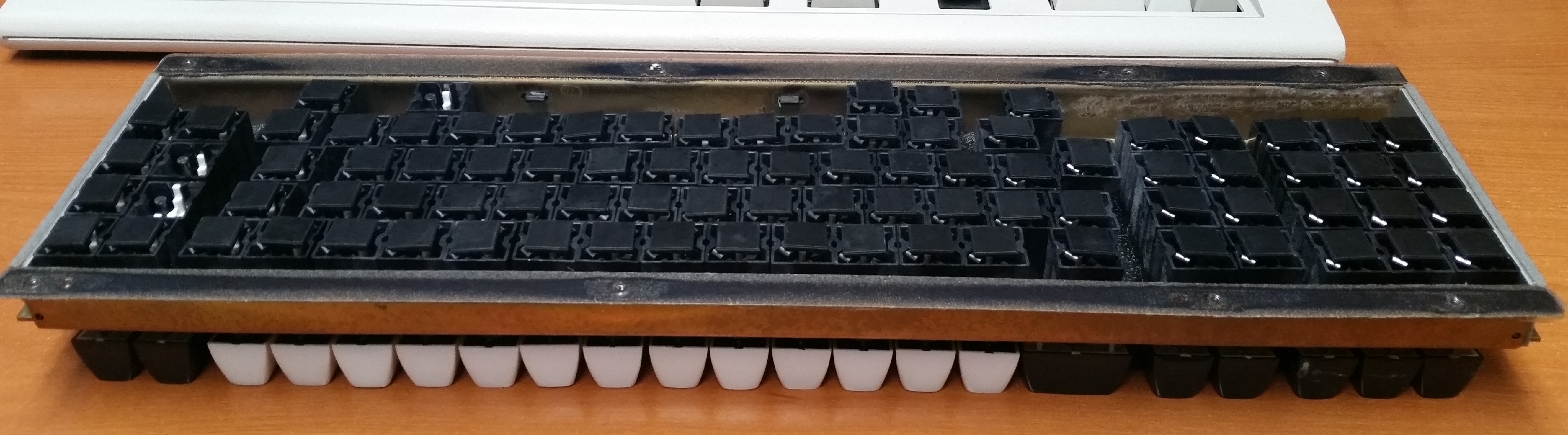This close-up photograph showcases the intricate inner workings of a keyboard that's been partially disassembled. The base of the keyboard has been removed, exposing numerous black plastic squares where the keys link into. These black squares are arranged methodically, akin to a typical computer keyboard, but notably devoid of any letters or numbers. Surrounding these black squares, we observe a framework accented with silver metal, which includes rivet holes presumably for screws or rivets. Alongside this, a thin piece of wood lines the outer front edge of the keyboard, giving it a distinct, elegant touch. The white and black keys are set against a light wood table, creating a contrasting background. Additionally, at the top section of the image, there's a glimpse of another white keyboard where the edges of its keys have gray, white, and black hues. The sight is further enriched by visible metal structures running along the insides and back of the keyboard, hinting at the sophisticated engineering behind it.